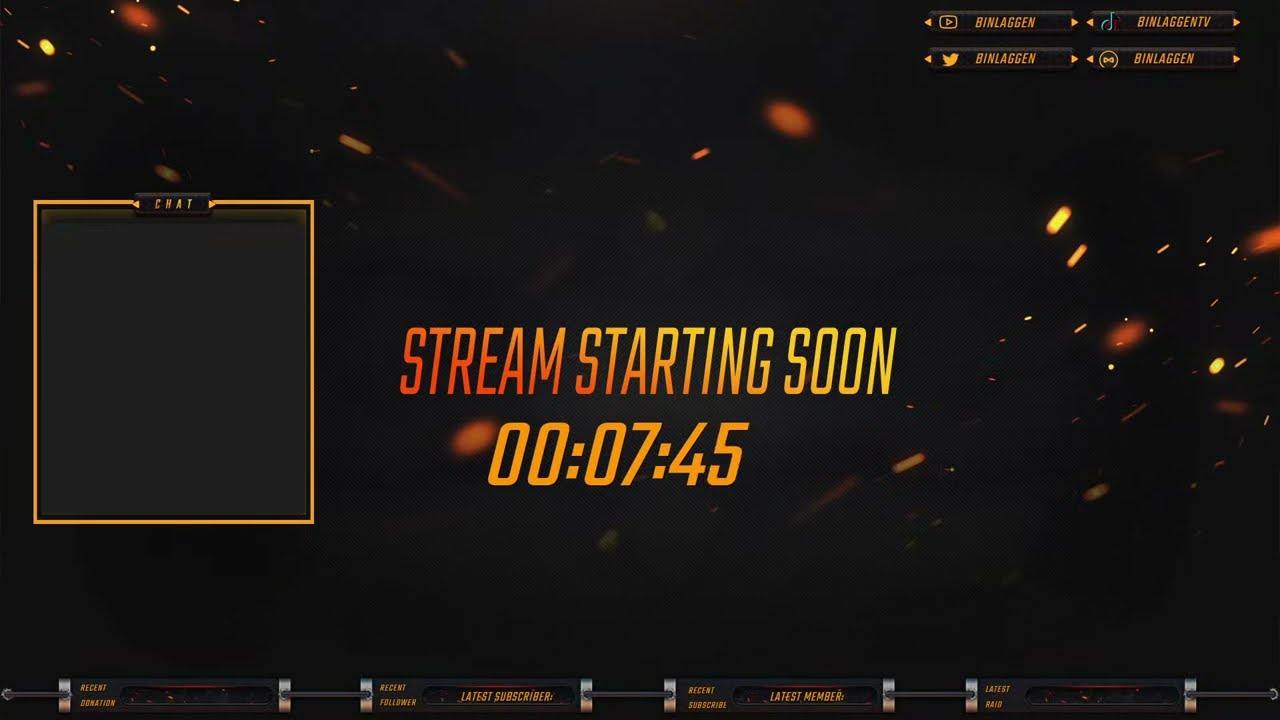The image is a horizontal rectangular splash screen for a video streaming service, showcasing the streamer's pre-live session. The background is predominantly black, evocative of outer space, filled with floating yellow and gold stars, creating an impression of embers kindling in the dark. Dominating the center of the screen are the words "STREAM STARTING SOON" in a gradient of red to yellow, with a countdown timer below reading "00:07:45" in bright, pale gold lettering, indicating the stream will begin in 7 minutes and 45 seconds. 

In the top right corner, small yellow text lists various social media handles, including Twitter, TikTok, and YouTube, all under the username "Binlaggen." Additionally, a yellow-outlined square sits to the left of the main text, with the word "chat" in yellow, though no one is currently in the chat. At the very bottom of the screen, there are white columns of text, likely saying "latest member," but they are too small to discern. This setup clearly prepares viewers for the upcoming live stream, providing a cohesive and visually engaging waiting screen.